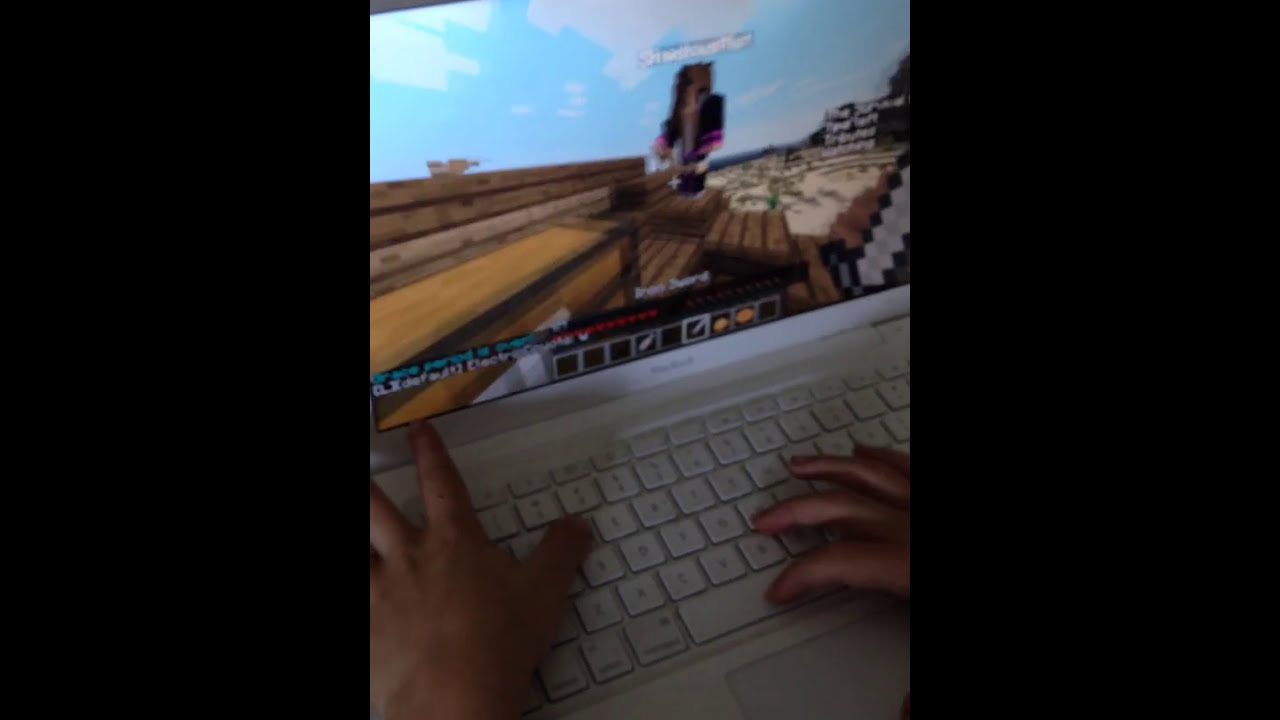In this dimly lit photograph taken from a slight angle above and to the left, we see a close-up of a white laptop, possibly a MacBook Pro, with a pair of olive-skinned hands positioned on the keyboard. The left hand is closer to the screen while the right hand hovers near the spacebar. The laptop screen displays a pixelated game interface, unmistakably reminiscent of Minecraft. The game setting shows an outdoor world with elements like a blue and white sky, brown wooden crates, and what seems to be sand in the background. A Minecraft character, wearing a black jacket, stands on these crates with white text above them, though it's too blurry and low-resolution to read. In the bottom right corner of the screen, a large sword icon suggests the player is either building something or engaged in combat.